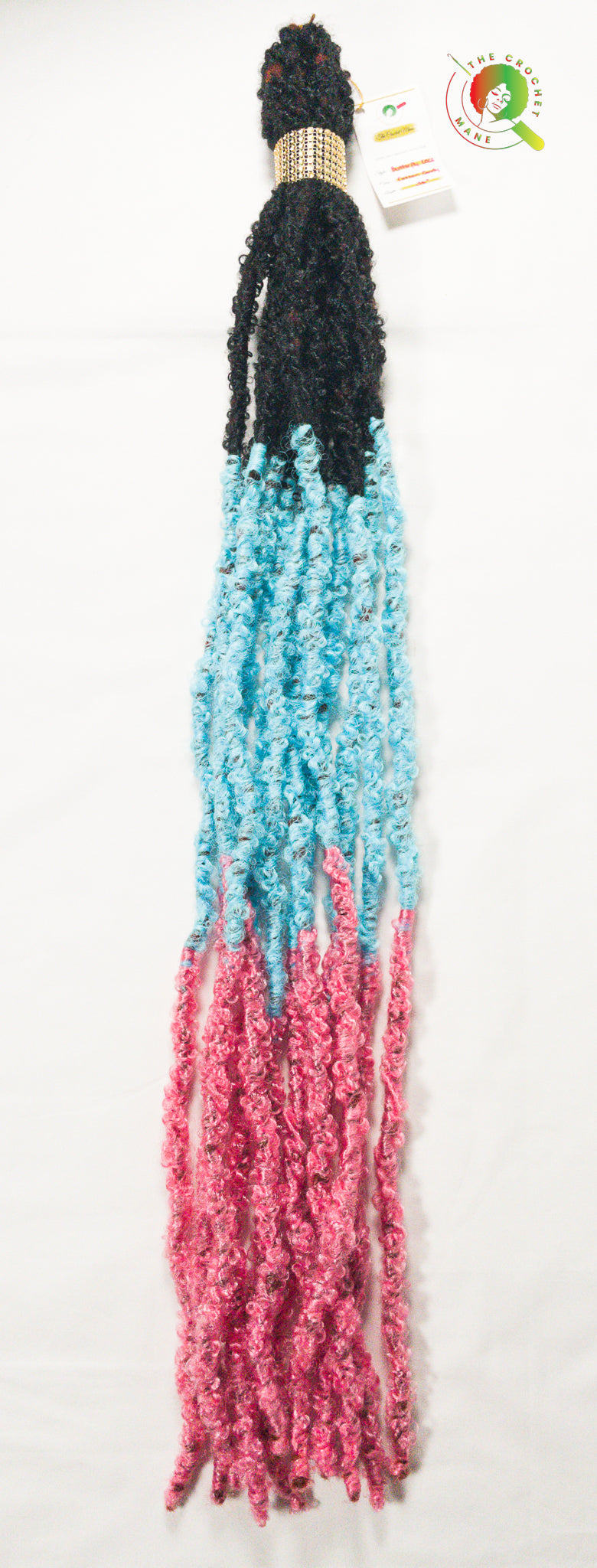The image depicts a decorative hair ornament designed to resemble long, colorful strands tied together at the top with a golden band. The ornament is constructed from a yarn-like material, featuring three distinct color sections: black at the top, transitioning to light blue in the middle, and ending with red at the bottom. The strands appear slightly wavy and flow vertically along the length of the ornament. Attached to the top is a small white tag with red and yellow lettering, alongside a circular emblem displaying the logo of the manufacturer, which seems to read "The Crochet Mane." The ornament is laid out on a white table, within a vertical rectangular photograph, and measures approximately 12 to 16 inches in length.